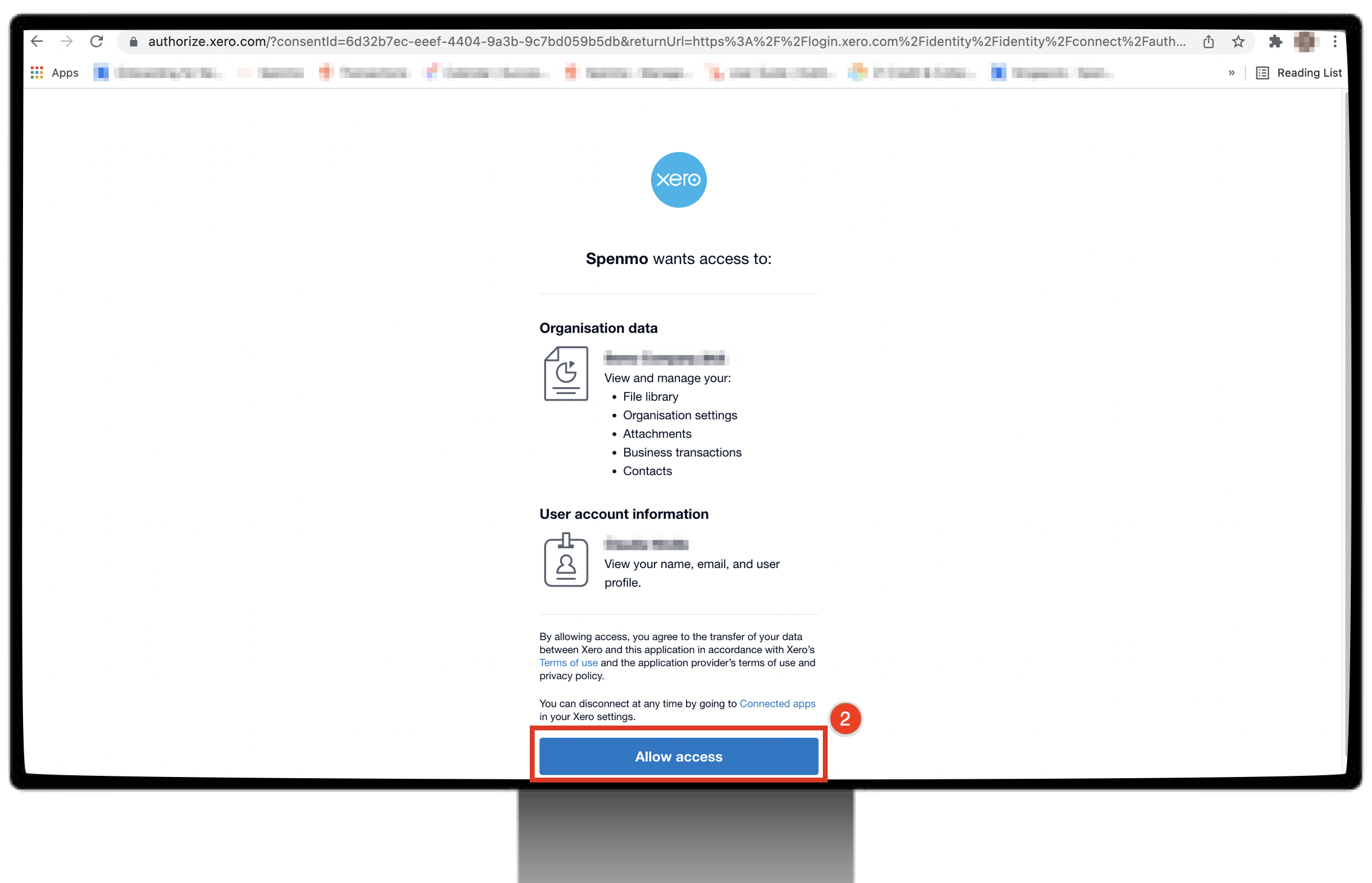A highly detailed mock-up of a website screen is depicted, designed to simulate a large flat-screen computer monitor. In the top-right corner, a user’s profile picture is visible, though it appears pixelated and grainy. Central to the image’s layout, the browser bar displays an extensive URL, and beneath it, a list of bookmarks, which are also obscured by pixelation.

Dominating the middle of the screen, a blue logo introduces a section that reads, "Spinmo wants access to." Below this header, a centered list itemizes specific permissions: the first item under "organization data" and under "user account information" are both pixelated. This suggests that sensitive details are being redacted.

At the bottom center of the screen, a prominent blue rectangle button labeled "Allow Access" in white font stands out. Encircling this button, a red box is highlighted, emphasizing its importance with a red number "2." This corresponds with a small red circle in the top-right corner bearing a white number "2," indicating that this represents step two in a series of instructions.